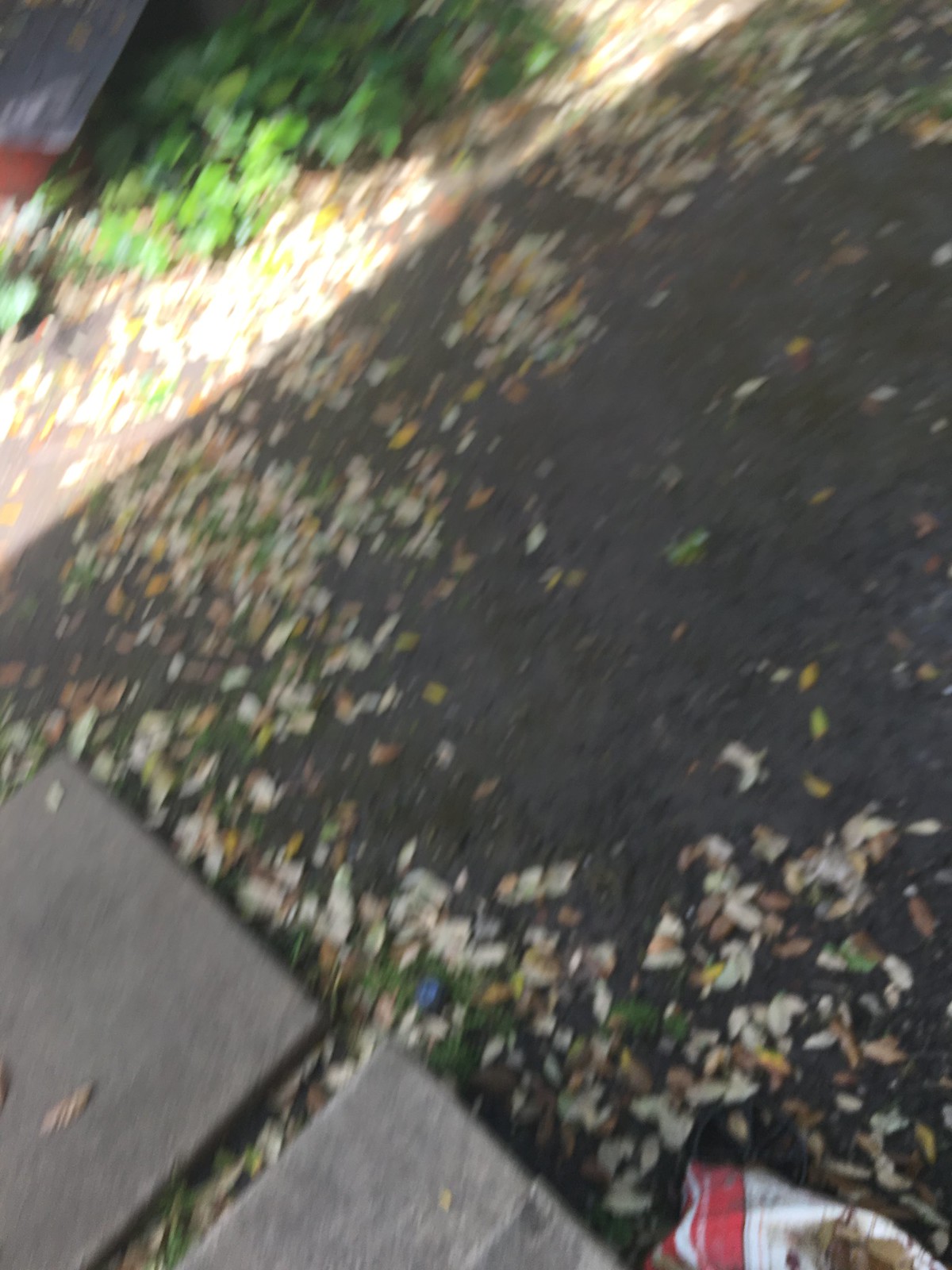The photograph appears slightly out of focus and may have been taken accidentally, capturing a shaded dirt pathway scattered with dry, broken leaves forming a rough U shape. In the lower right corner, a somewhat crumpled white and red bag, possibly once containing potting soil, is visible. The path features two concrete stepping stones set apart from each other, suggesting they might be used to traverse the area when it becomes muddy. On the upper left, a bed of greenery and a bush can be seen, partially overlapping with a bright sunlit strip cutting across the ground from left to right. Nearby, the path appears compacted, hinting at either dark cement or well-trodden dirt, with occasional clumps of grass and a few large green leaves adding texture to the scene. The presence of an unclear object, possibly the corner of a car or a toolbox, further adds to the ambiguity of this blurry outdoor snapshot.